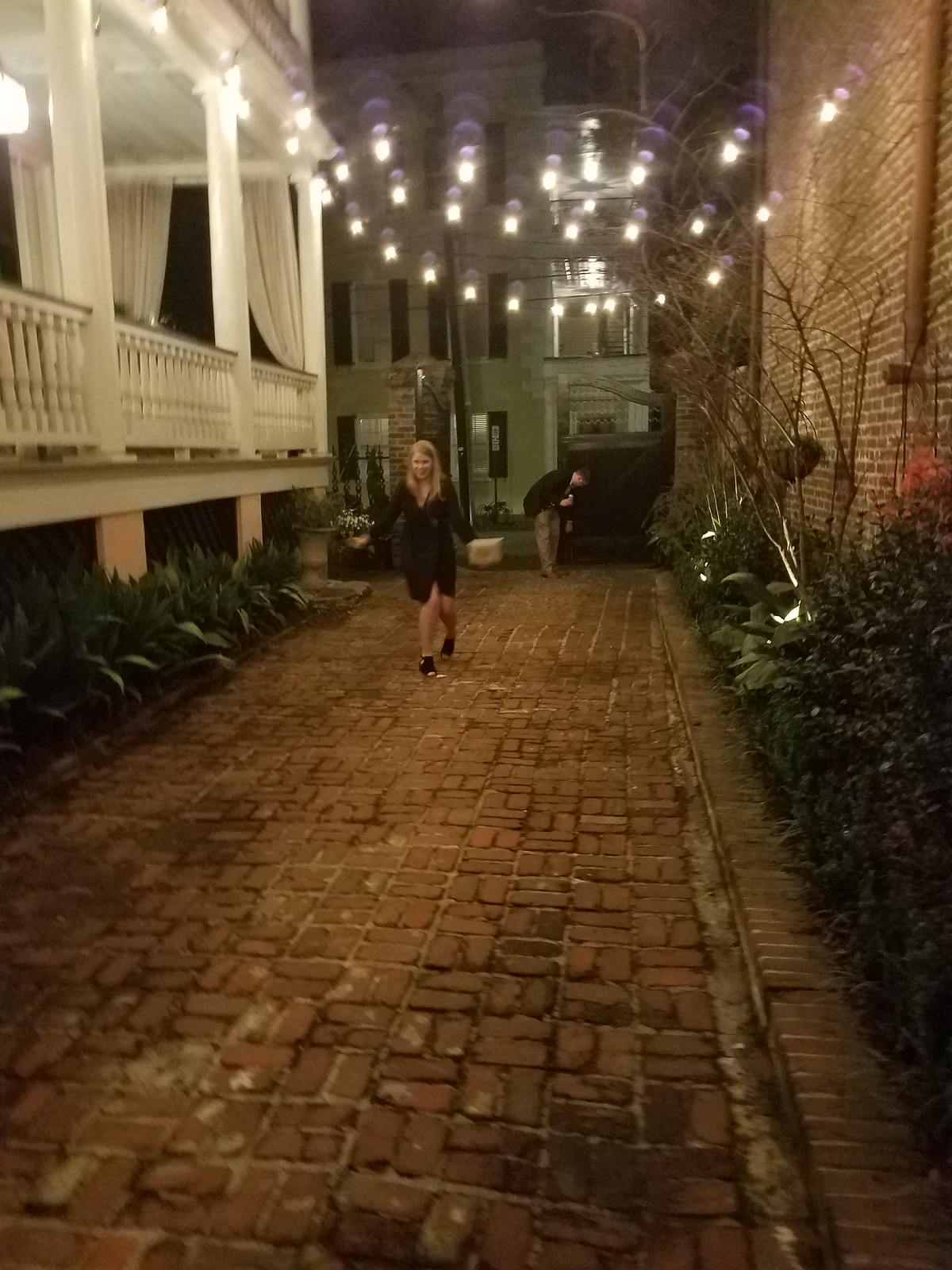In this picturesque urban scene, a narrow brick-paved alleyway winds between a solid brick building on the right and a house with a prominent white balcony on the left. The intricate arrangement of little bricks on the ground adds a rustic charm, contrasting with the modern string lights that arch overhead, connecting the two structures with three delicate strands. A lone woman dressed in an elegant black dress makes her way down the path, moving towards the viewer with an air of quiet contemplation. 

On either side of the walkway, patches of green shrubbery offer a touch of nature amidst the urban setting. The white balcony on the left side stands out, adorned with graceful curtains and softly glowing lights, creating a cozy, welcoming atmosphere. Higher up from the balcony, there is an expansive porch that further enhances the house's charm. 

In the distance, a gray building marks the end of the walkway. Near this building, a man is slightly bent over, perhaps attending to something on the ground. The overall ambiance is serene and inviting, capturing the essence of a quiet, lovely moment in a bustling city.